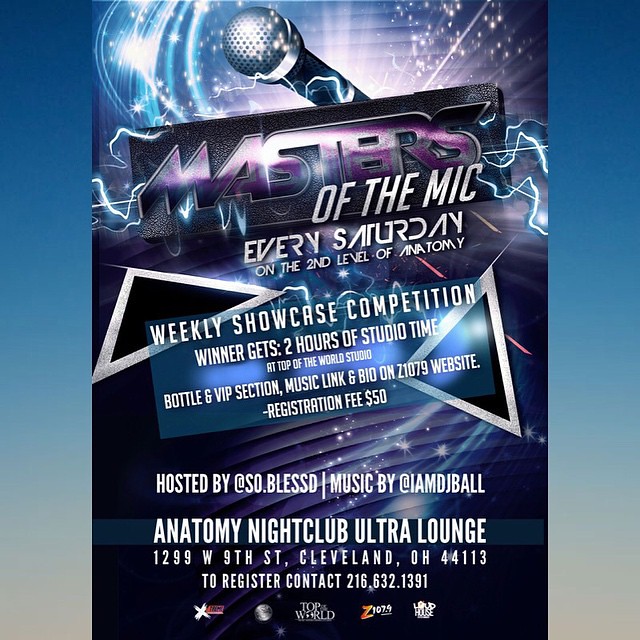The image is a promotional poster featuring a vibrant and electric backdrop. At the top, dark-blue and light-blue swirls mixed with purple hues and sparkles complement a darker sky transitioning to gray at the bottom. Central to the scene is a microphone angled forward, surrounded by lightning bolts emanating from the word "Masters" written in a striking multicolored purple and black font on a black background. Below "Masters," it declares in white text: "of the MIC," followed by "Every Saturday" and "on the second level of Anatomy."

Beneath these headlines is a light-blue banner adorned with metallic-looking triangles. The banner proclaims in white: "Weekly Showcase Competition. Winner gets 2 hours studio time at Top of the World Studio. Bio and VIP section, music link and bio on Z1079 website. Registration fee, $50."

At the bottom, the poster lists further details: "Hosted by @soul.blessd. Music by @iamdjball," accompanied by contact and venue information: "Anatomy Nightclub Ultra Lounge, 1299 West 9th Street, Cleveland, Ohio 44113. To register, contact 216-632-1391."